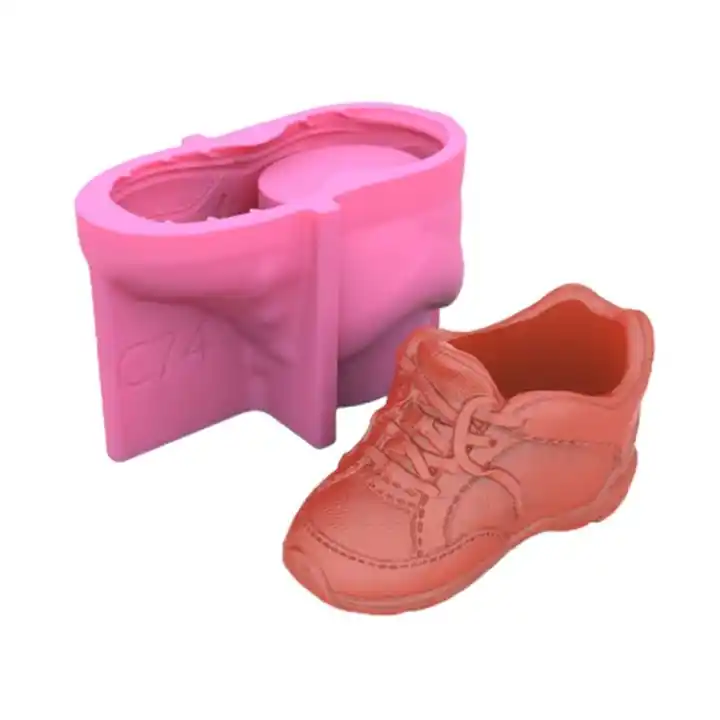The image depicts a small, detailed brown-bronze colored shoe, resembling a traditional baby shoe, positioned beside its corresponding mold. The shoe, which appears to be made from either plastic, wax, or a clay material due to its smooth, consistent texture and reflective surface, features intricate details including untied laces, visible stitching, and a hollow interior. It resembles an old-fashioned sneaker complete with a discernible edge along the sole. The mold, appearing to be made from a pink silicone material, lies upside down to the top left of the shoe. The underside of the mold reveals the cavity that shapes the sole of the shoe and is marked with the inscription "C-74" in the bottom left corner. Both the shoe and the mold are placed against a pristine white background, highlighting their contrasting colors and textures.